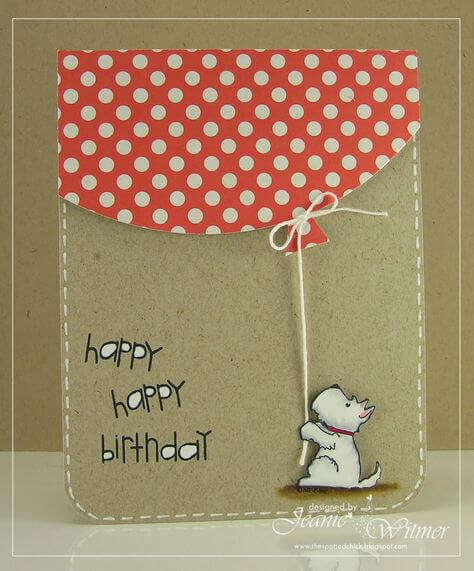A full-color photograph captures a creatively designed birthday card positioned against a brown wall and a white countertop, surrounded by a white border. The card features a playful layout with the phrase "Happy Happy Birthday" in a whimsical font located at the lower left-hand corner. On the lower right, it is marked as "designed by Jeanne Whitmer."

The card's central illustration showcases a small, cute white dog holding onto an actual string that is attached at the bottom. The string extends upwards to the flap of the envelope, which is cleverly designed to resemble a red balloon with white polka dots. The card itself appears to have a light brown, cardboard-like texture and is accented with white stitches around the edges, giving it a handmade, craft-project feel.